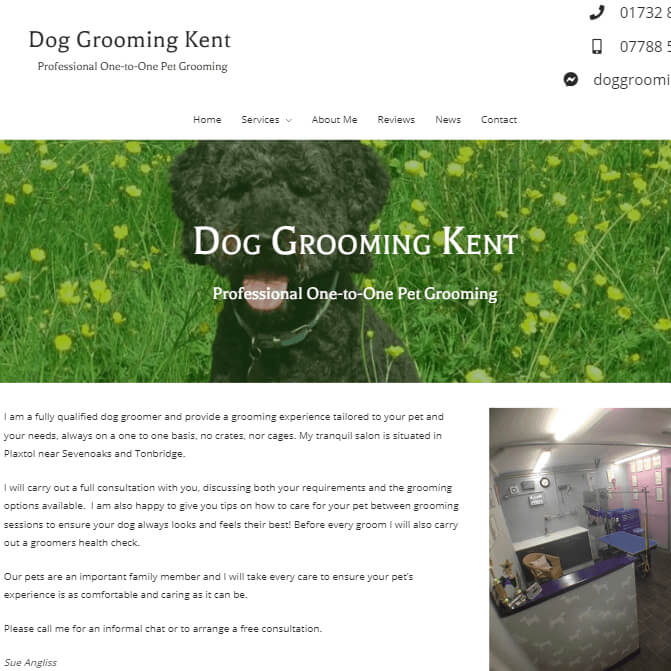The image showcases a website for a dog grooming business located in Kent. In the top left corner, bold black text announces "Dog Grooming Kent," followed by a smaller text that reads, "Professional One-on-One Pet Grooming." Adjacent to this, on the right, there are contact icons: a telephone symbol with a partially visible number "01732," a mobile phone icon displaying "07788" with part of the number cut off, and a Facebook message button indicating "DOGGROOM" with the rest truncated.

Beneath the header, navigation tabs are listed from left to right: Home, Services (with a downward-facing arrow), About Me, Reviews, News, and Contact, all in black.

Dominating the center of the page is a rectangular image featuring a lush green field dotted with yellow flowers. In the foreground, a fluffy black dog pants happily, tongue peeking out, wearing a green collar. Superimposed on this image, white text repeats the business name "Dog Grooming Kent" and the tagline "Professional One-to-One Pet Grooming."

Below this image, black text on the left-hand side provides detailed information about the services:
 
"I am a fully qualified dog groomer and provide grooming experiences tailored to your pet and your needs, always on a one-to-one basis. No crates, no cages. My tranquil salon is situated in Plaxtol, near Seven Oaks and Tonbridge. I will carry out a full consultation with you, discussing both your requirements and the grooming options available. I am also happy to give you tips on how to care for your pet between grooming sessions to ensure your dog always looks and feels their best. For every groom, I will also carry out a groomer's health check."

Further down, additional text emphasizes the personal care aspect: "Our pets are an important family member, and I will take every care to ensure your pet's experience is as comfortable and caring as it can be."

Toward the bottom, it encourages potential clients to reach out: "Please call me for an informal chat or to arrange a free consultation." This segment ends with the signature, "Sue and Gliss," all in black text.

On the right side of the page, an image depicts the salon interior. The foreground features a counter with a black top adorned with pictures of dogs. The background reveals a grooming table and additional grooming stations.